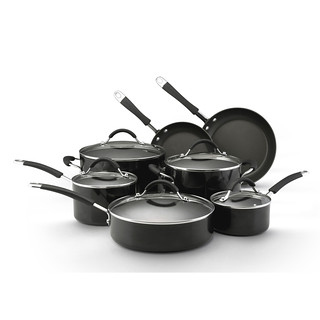This promotional image from a homeware catalogue showcases a stylish and versatile seven-piece cookware set, perfect for modern kitchens. The set includes five saucepans and two frying pans, all crafted in a sleek dark grey, almost black hue. The saucepans come with see-through glass lids accented with black handles and silver rims, securely fastened with screws. Each piece has well-designed, curved handles providing ample space between the handle and the lid to ensure safe handling. The two frying pans—one larger, the other smaller—are positioned in the background with their handles protruding to the left. The saucepans vary in size and shape, with three featuring long handles for easy maneuvering and two substantial pots having dual side handles for safe lifting. Notably, while the casserole pots with side handles can't be hung, the rest of the pots have hanging capabilities, adding convenience for kitchen storage. The set is professionally arranged in front of a white background, emphasizing its modern and functional design, making it ideal for catalog advertising.